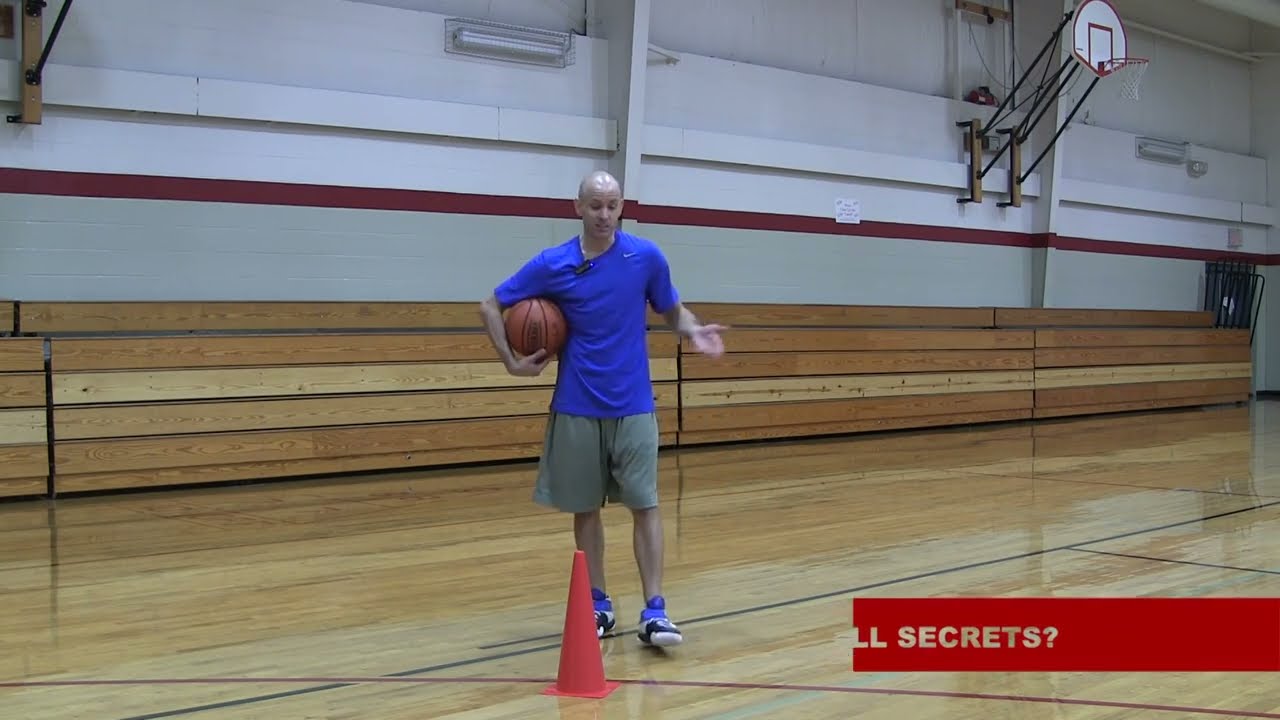The image depicts a bald man with a shiny head standing on an indoor basketball court. He is wearing a bright blue short-sleeve t-shirt, light gray shorts, and bright blue and navy blue sneakers with white accents. The man, who is holding a basketball with both hands below his chin, is positioned near an orange cone on the court's hardwood floor. The gym's walls are white with a red stripe and made of wooden panels, with bleachers folded up against the wall. On the right side of the image, you can see an entryway with bars above it. A basketball hoop is visible in the upper right corner, pulled upwards to make way for the bleachers. The setting suggests the man is preparing for or demonstrating a basketball move.